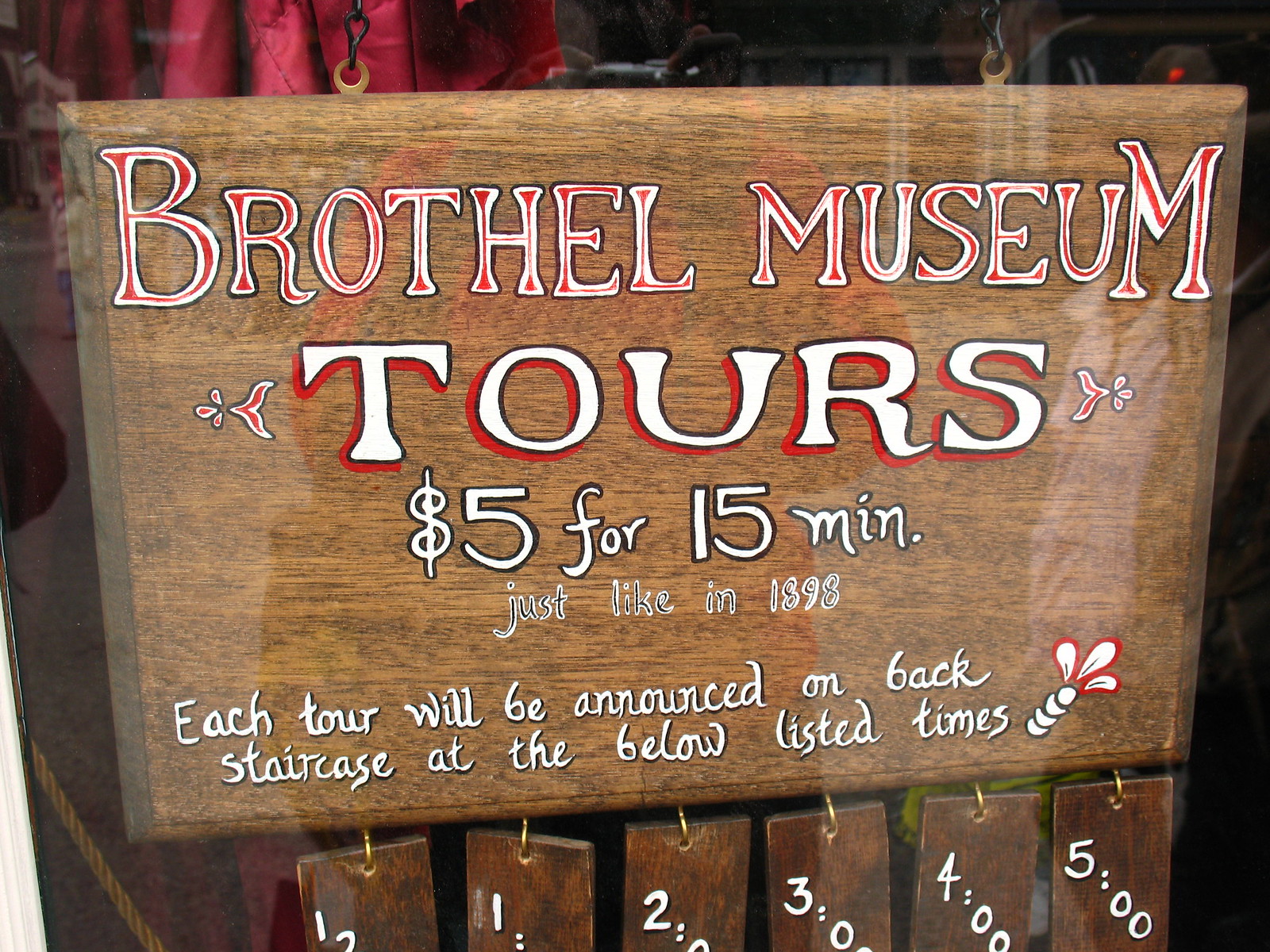The image features a wooden sign with prominent, old-style red and white lettering, advertising the "Brothel Museum." The title "Brothel Museum" is in bold white with red outlines. Below, "Tours" is highlighted in red and white, followed by the text: "$5 for 15 minutes just like in 1898." Further down, it states, "Each tour will be announced on Back Staircase at the below listed times," elucidating the tour times as 12 o’clock, 1 o’clock, 2 o’clock, 3 o’clock, 4 o’clock, and 5 o’clock. Six numbered tags hanging from brass hooks on the bottom of the sign display these times. The sign is situated behind a window with noticeable reflections of people observing it. A partially open curtain, deep red or burgundy in color, is visible to the left-hand side of the image, inside the store.